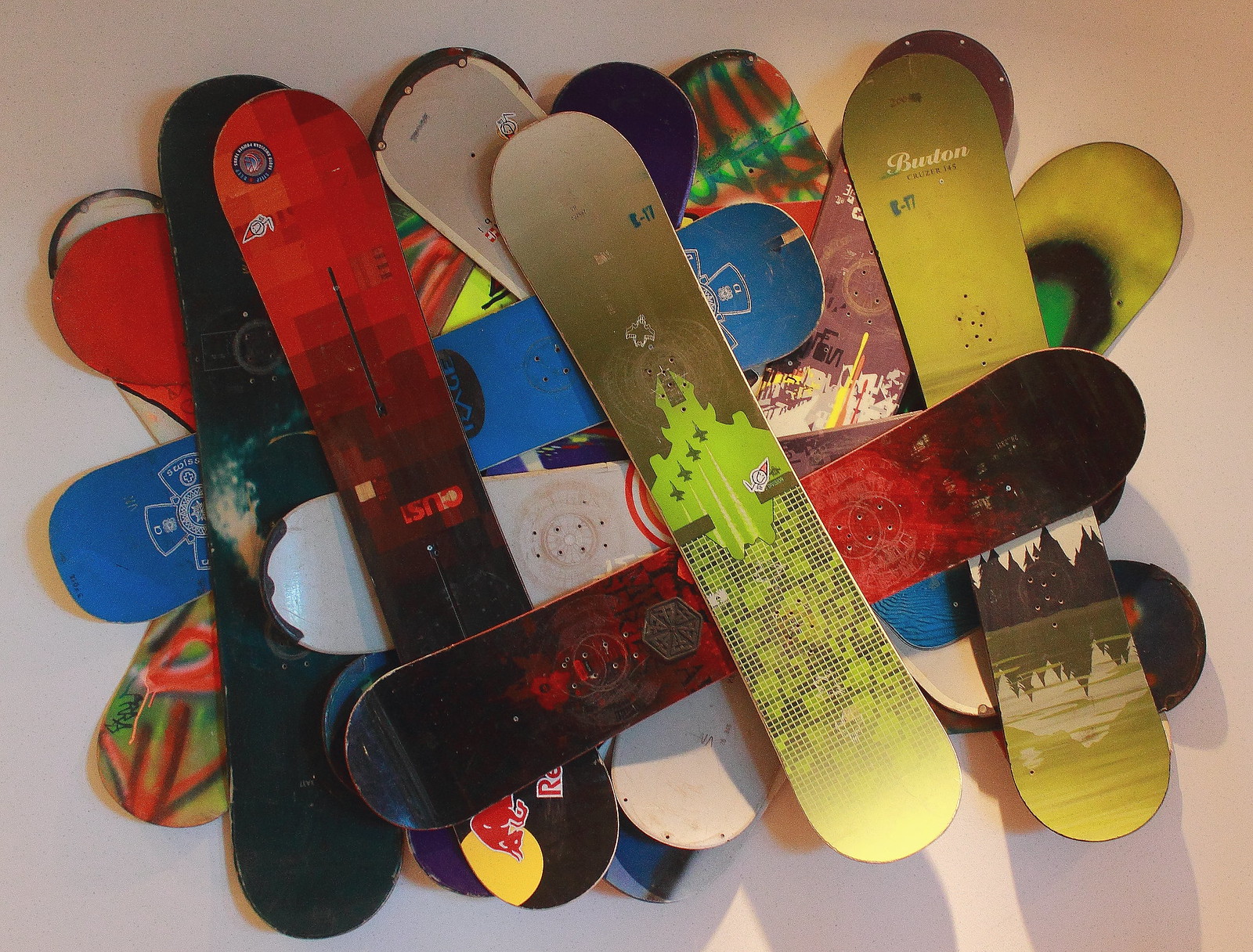In this photograph, a chaotic yet intriguing pile of snowboards lies sprawled across a beige-white surface, with the warm lighting casting a beige hue over the setting. The snowboards create a lattice-like pattern due to their varying orientations, some being more vertical and others more horizontal. There are approximately 15 to 20 snowboards, layered about four deep, showcasing a kaleidoscope of colors and designs. Prominently visible are snowboards with red, green, yellow, teal, and black-and-red designs. The green design features airplanes, reminiscent of a military theme, while another board displays a tie-dyed pattern. Among the brands seen is a Burton snowboard with variations of green and mountain imagery, and potentially a K2 board. The ends of the snowboards curve upward, adding to the dynamic and haphazard arrangement. Shadows cast by the photographer are noticeable in the background of the image.